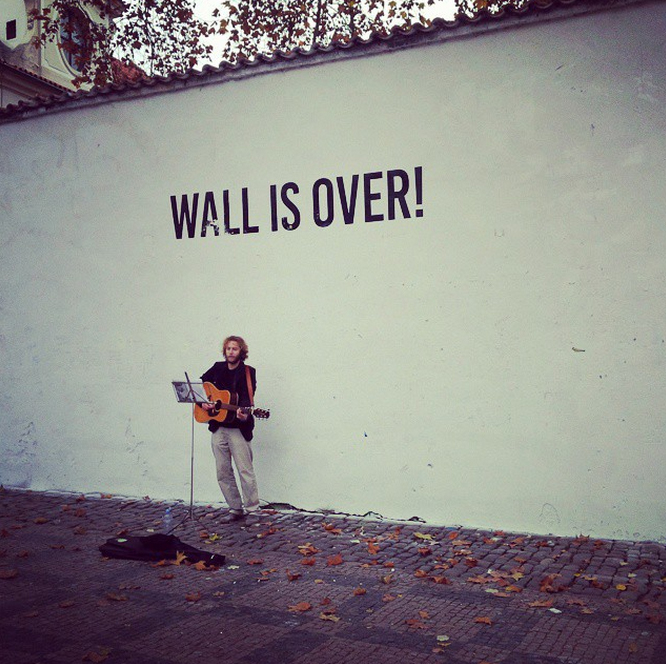The image depicts an outdoor acoustic set featuring a man with blondish-brown hair, some facial hair, and dressed in white pants and a dark top. He is standing in front of a large, white-ish wall adorned with the purplish text "Wall is over!" followed by an exclamation point. The man plays a standard brown acoustic guitar with a brown strap and performs from a metal music stand holding sheet music. At his feet lies an open guitar case, though its contents are not visible. The pavement beneath him consists of a textured pattern resembling individual pavers or bricks, forming squarish outlines in darker shades that could be black or dark burgundy. Surrounding the scene, reddish-leaved trees drop leaves scattered across the pavement, adding a mix of orange and brown hues to the environment. Off to the left in the background, the top of a house with its roof and window can be seen, contributing to the ambiance of a street or neighborhood setting.